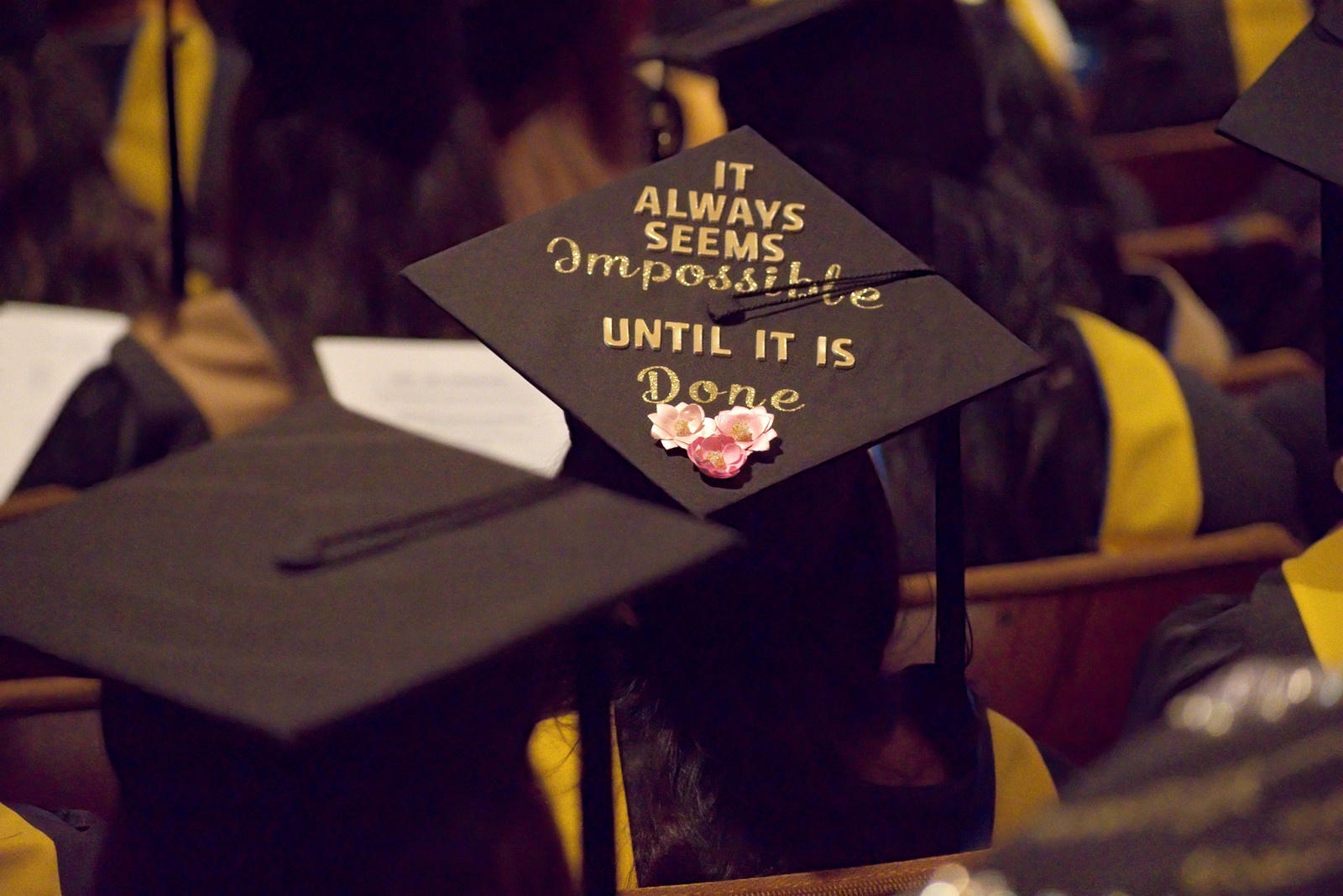This photograph captures the backs of graduating students seated in wooden benches, wearing black gowns with yellow sashes draped over their shoulders. Each student sports a graduation cap with the tassel hanging to the right. Central to this image is one distinctive cap adorned with gold embossed writing. The text, in part cursive, reads: "It always seems impossible until it is done," followed by three pink flowers. The contrast of the black and yellow attire against the subtle details of the decorated cap draws focus, encapsulating the celebratory essence of the graduation ceremony.